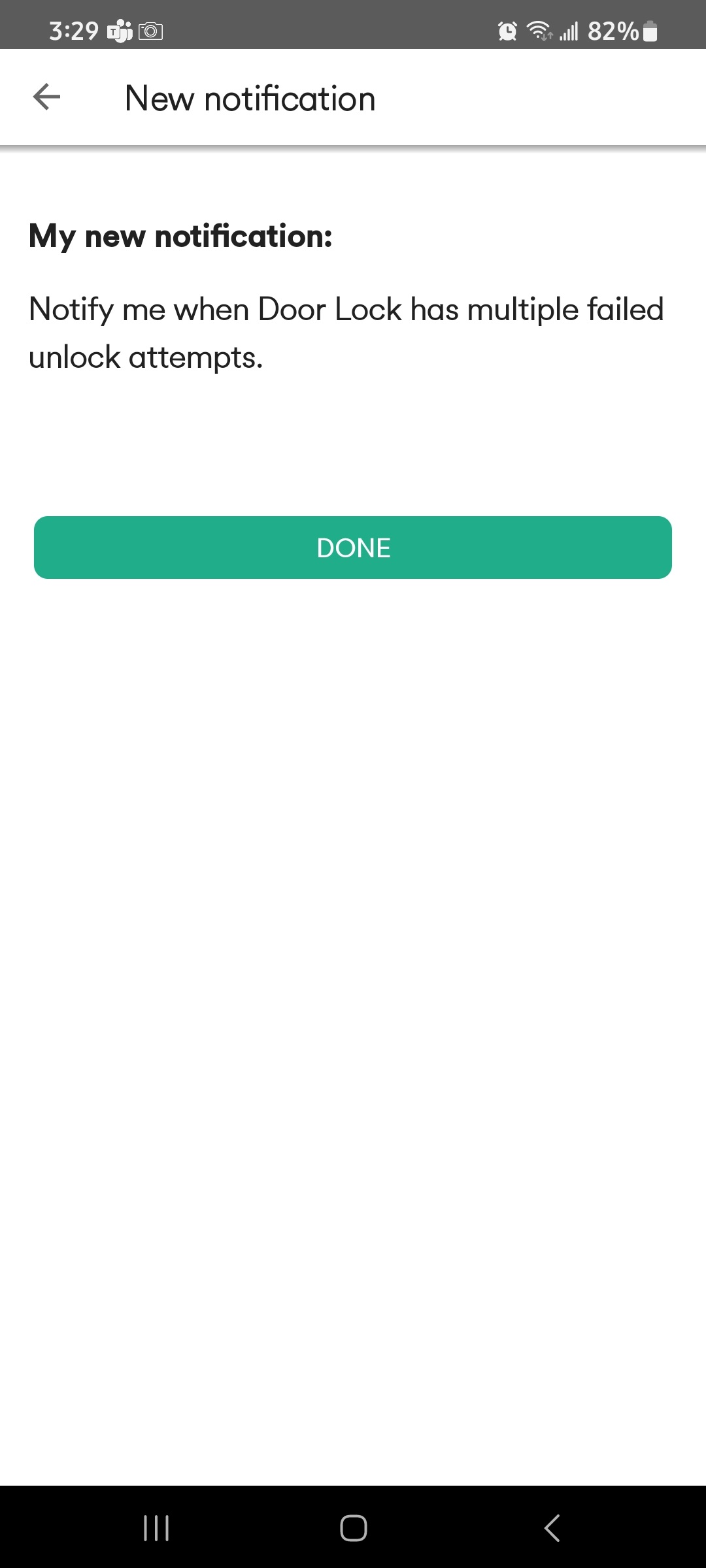This image, captured from a cell phone screen, shows a comprehensive view of a notification interface. At the top of the screen, there's a gray status bar. On the left-hand corner of this bar, the time is displayed as "3:29." Adjacent to the time, there are two icon symbols, followed by a considerable blank space. To the right of this space, there are three to four additional icons, indicative of various notifications or statuses. Further to the right, the battery status is indicated at "82%" with a white battery icon, next to which is a downward-facing arrow.

On the left side below the status bar, there's a left-pointing arrow accompanied by the text "New Notification." This section is demarcated by a light gray line running horizontally across the screen. Directly under this line, the text reads: "My new notification: Notify me when door lock has multiple failed unlock attempts." 

Below this notification message is a green button that reads "Done." The background in this section is entirely white and unadorned, giving it a clean, uncluttered appearance. Towards the bottom of the screen, a black rectangle contains navigation icons: three horizontal bars, a circle, and an arrow.